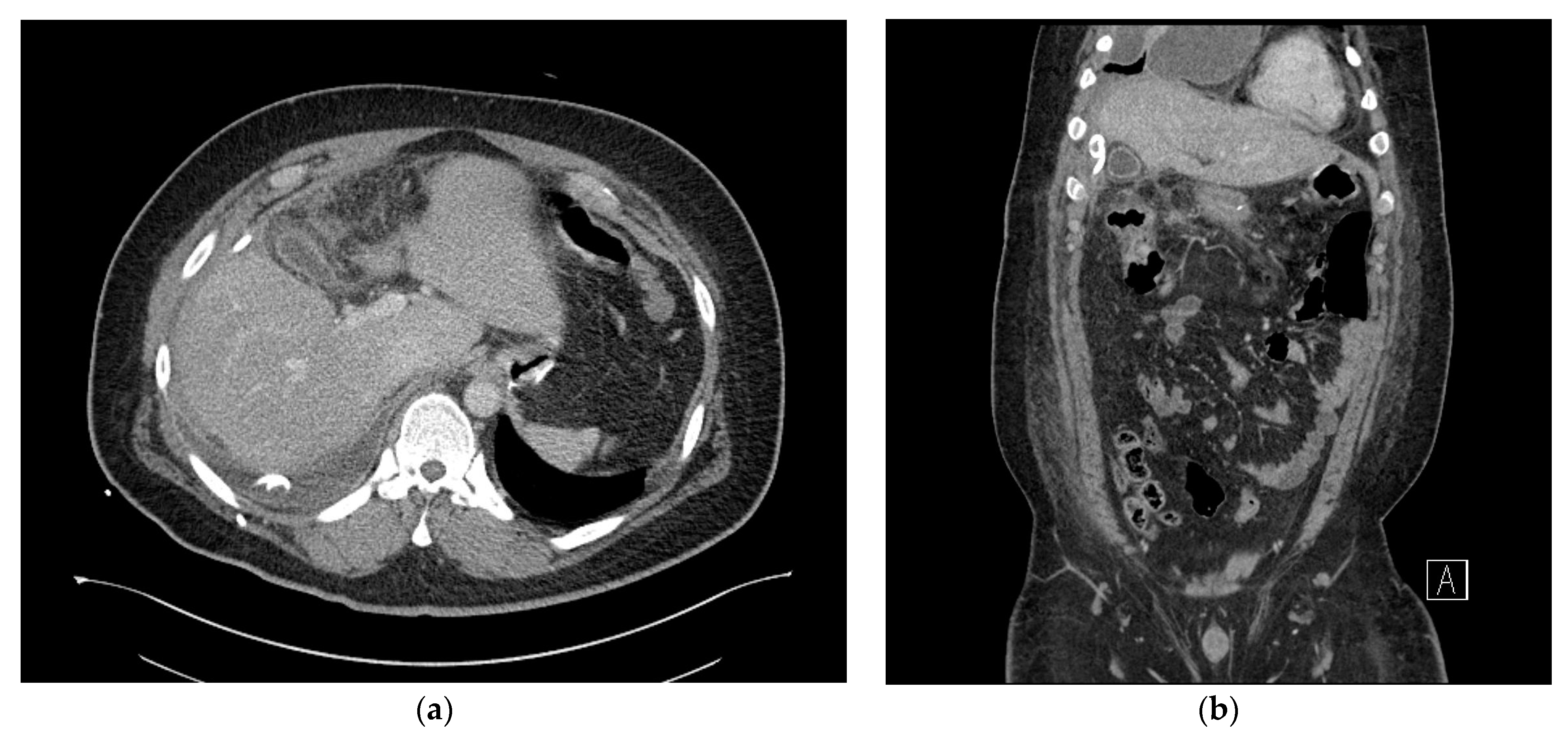This set of two medical scans, captured in black and white x-ray or MRI format, provides distinct perspectives on anatomical structures. On the left, image A showcases a side view of a head, likely a brain x-ray, outlined with a bright, chalk-like line and featuring various shades indicating different brain regions. There are noticeable white spots and darker shaded areas, although it is unclear if the darker shading represents the front or the back of the brain. On the right, image B presents a top or bottom view of an anatomical structure, heavily shaded with a mix of dark grays and blacks. The most striking features include rows of bright white spots near the top, possibly rib cross sections, and other vague shapes suggestive of internal organs. This scan also contains evenly spaced white dots along the edges. While some aspects of image B's anatomy remain ambiguous, there is speculation it could represent a torso or another cross-section of the body, potentially even of an animal due to the unclear overall shape and presence of what might be limbs or toes at the image's top.